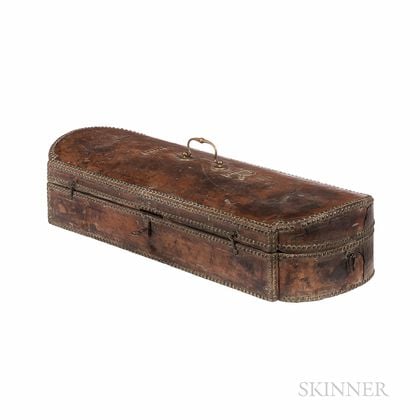This image is a color photograph of a long, oval-shaped leather case. The case is quite narrow, with flat sides and curved ends, resembling a narrow casket or a case for an instrument like a violin or a guitar. The exterior is made of brown leather that appears to be in rough shape, possibly deteriorating. On the front side of the case, there is a key sticking out of a lock mechanism, indicating it can be securely closed. A small metal handle at the top allows it to be carried. The case also features two metal buckles or hooks. The background is plain white, and in the bottom right corner of the image, the word "Skinner" is clearly visible in gray text. The case’s distinctive shape and features suggest it might be a specialized container, although its exact purpose remains unclear.